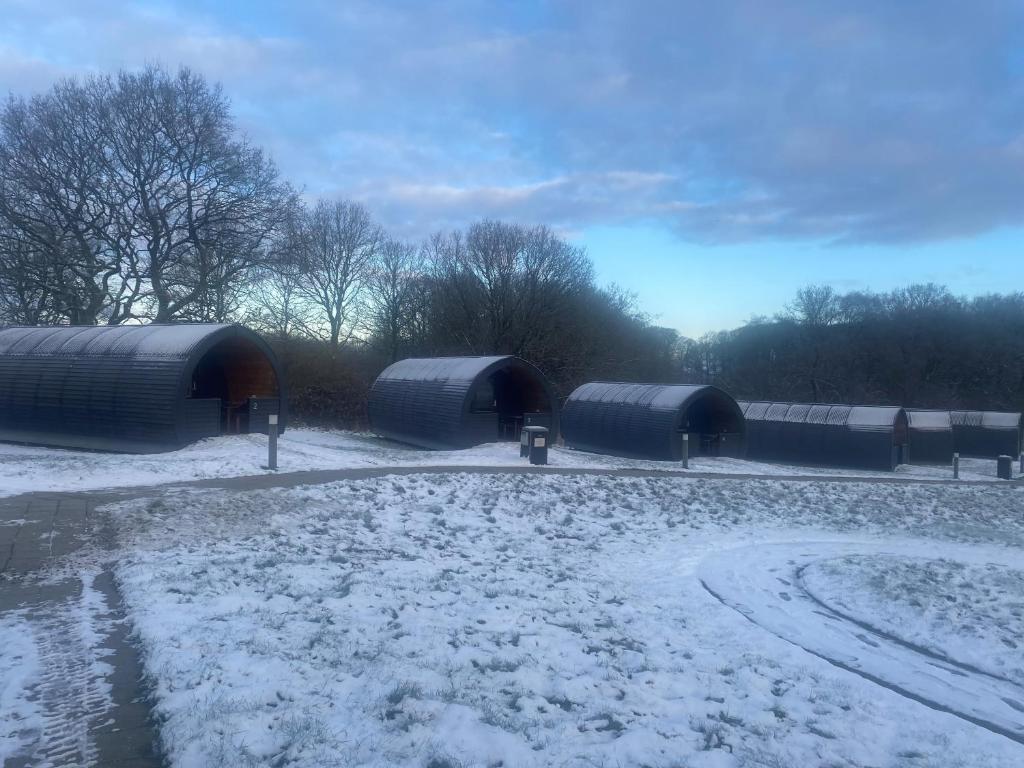The image depicts an outdoor winter scene featuring six half-circular, dome-shaped shelters that resemble military barracks or barns. These structures, characterized by their black siding and completely open fronts, sit in a snowy landscape. Each of the shelters appears to have a small door frame or gate at the bottom center of the opening. A dark roadway runs in front of these shelters, curving around them, with what looks like mailboxes or posts next to each building. The ground is entirely covered in snow, and a light dusting of snow is visible on top of the structures as well. Behind the shelters stand tall, leafless trees, adding to the wintery atmosphere. The sky overhead is a wintry mix of light blue and gray, with large clouds suggesting cold, overcast daytime conditions. The photo, taken from a standing vantage point, captures the stark beauty and tranquil stillness of the scene.